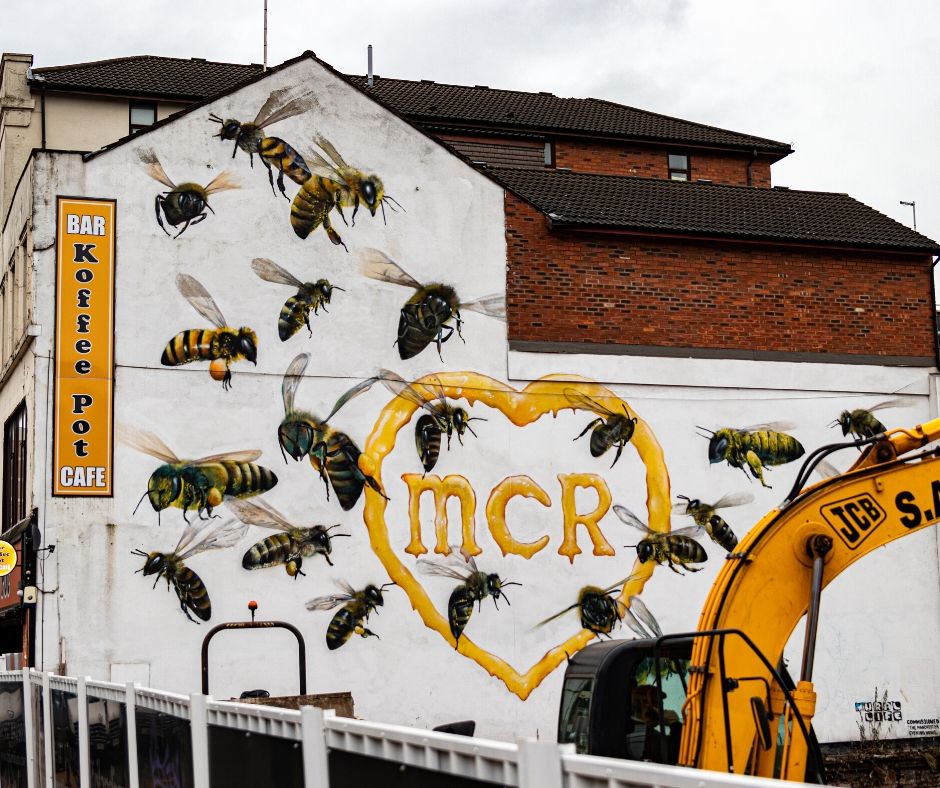This photograph captures the exterior side wall of a building, predominantly painted white with artistic mural features. The mural showcases numerous yellow and black butterflies scattered across the wall, with a central heart shape painted in yellow, containing the letters "MCR". On the left side of the mural, a vertical rectangle displays the words "Bar, Coffee, Port, Cafe." The building itself has a section constructed with brown-colored bricks, and it is topped with a dark brown roof. Also captured in the scene is a yellow and black JCB machine positioned outside the building. Overhead, the sky is adorned with clouds, adding a dynamic background to the vibrant mural and overall composition of the photograph.